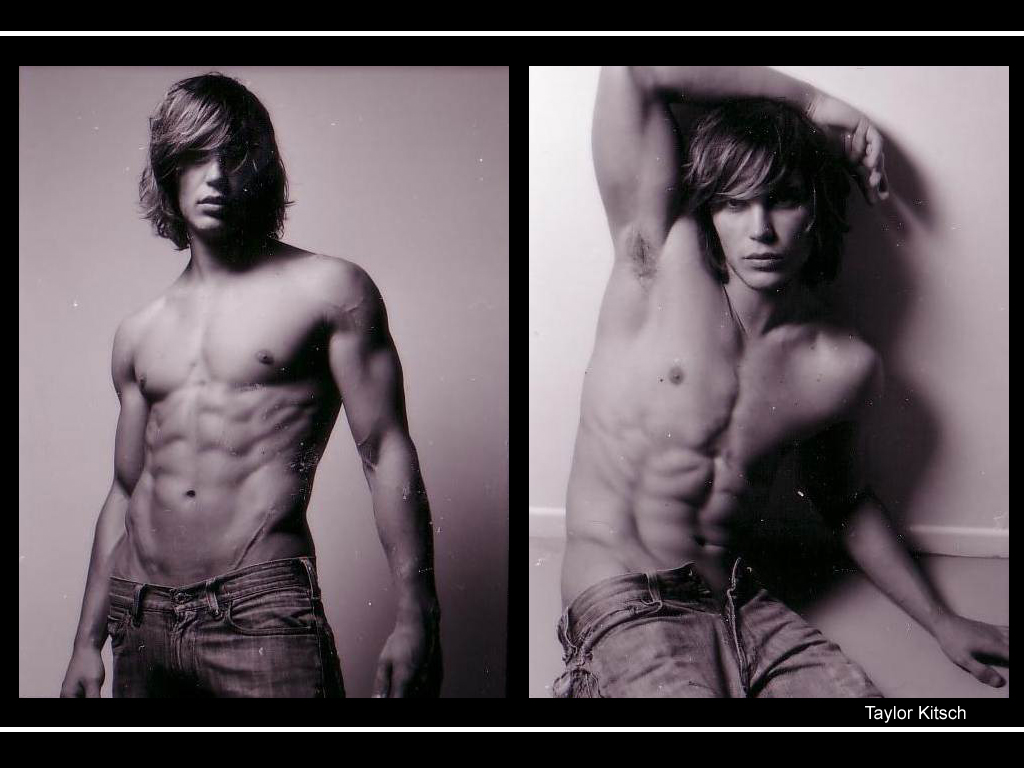In the image, there are two side-by-side black and white photographs of a male model, Taylor Kitsch, separated by a black divider. Both pictures feature Kitsch shirtless and wearing jeans. In the left photo, he is standing in a powerful stance, showcasing his defined six-pack abs. His hair, which is just past chin-length with side-sweeping bangs, adds to his strong, mysterious look. The background is plain white, emphasizing the model's form. The right photo portrays Kitsch sitting on the floor in a provocative pose, with his jeans unbuttoned and slightly pulled down. His arm is raised over his head, exuding a sexy, confident vibe. In both images, he maintains a consistent hairstyle, further enhancing the cohesiveness of the series.